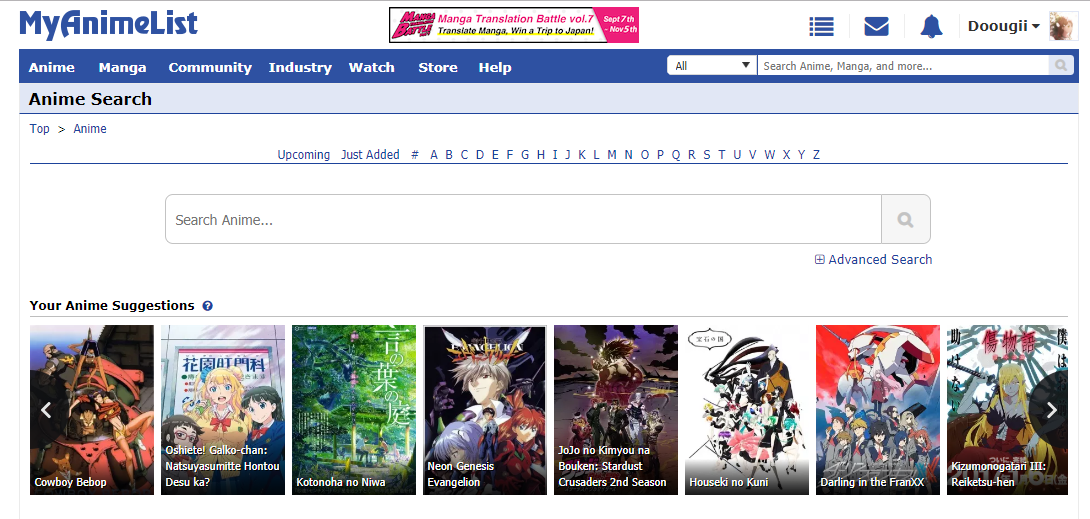The image shows a computer monitor displaying a logged-in MyAnimeList account. The interface features MyAnimeList's signature blue lettering against a white background. At the top right corner of the screen, the user "DuogiGuy" is logged in. Below the main MyAnimeList logo, there is a navigation tab bar with categories labeled: Anime, Manga, Community, Industry, Watch, Store, and Help. The current tab seems to be "Anime," specifically focused on the "Anime Search" section. The search input field is empty, awaiting user input. Below the search bar, there are eight anime movie suggestions listed, but the titles are too small to be legible. The interface also features sections for "Upcoming" and "Just Added" anime movies, sorted alphabetically from A to Z.